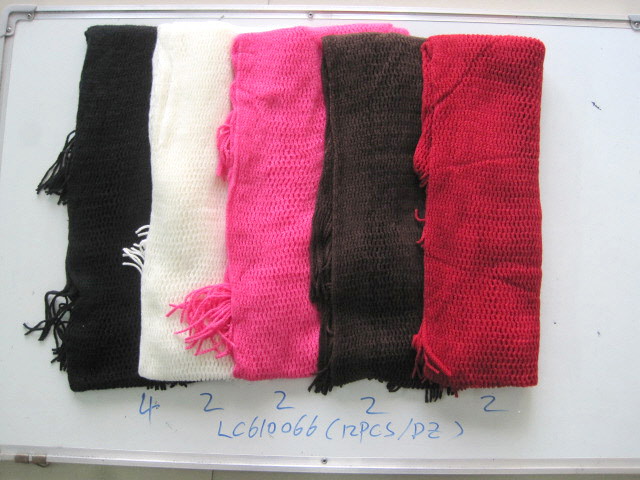This image features a detailed arrangement of five knitted scarves, each showcasing a soft, mesh-like weave and tassels at the ends. They're laid out horizontally from left to right, slightly overlapping one another. Starting from the left, the scarves are black, white, hot pink, brown, and bright crimson red. Each scarf has a corresponding number below it written on the whiteboard they are displayed on. The black scarf has the number 4, while each of the other scarves (white, pink, brown, and red) has the number 2 beneath it. Additionally, at the bottom of the whiteboard, there's a textual inscription in blue dry erase marker that reads "LC610066 12PCS/PZ." This comprehensive layout highlights the colors, texture, and organization of the scarves against the clean white background of the board.